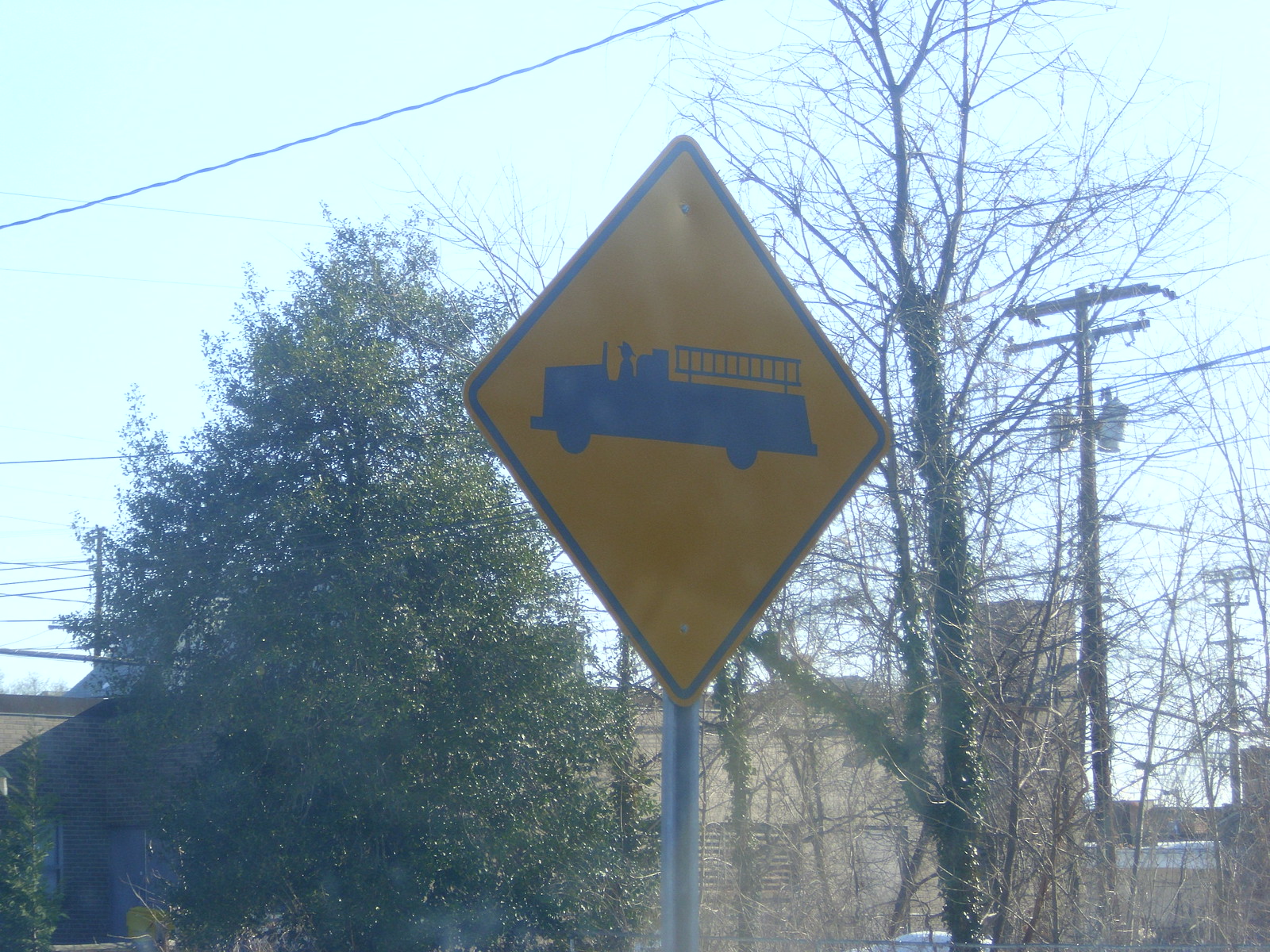This color photograph, likely taken from inside the passenger side of a car, features a slightly overexposed view of a city street. A minimal yet indistinguishable glare is present, adding to the aesthetic of the image. Dominating the center is a diamond-shaped street sign on a metal pole, dark yellow in hue, displaying a silhouette of a fire truck and a fireman. Behind the sign, urban elements, including buildings, trees, and a telephone pole on the right-hand side, are visible amidst the bright daylight. Tangled branches add an organic touch, and the play of light and shadows from the car window glass contributes to the overall atmosphere of a sunny, bustling city scene.